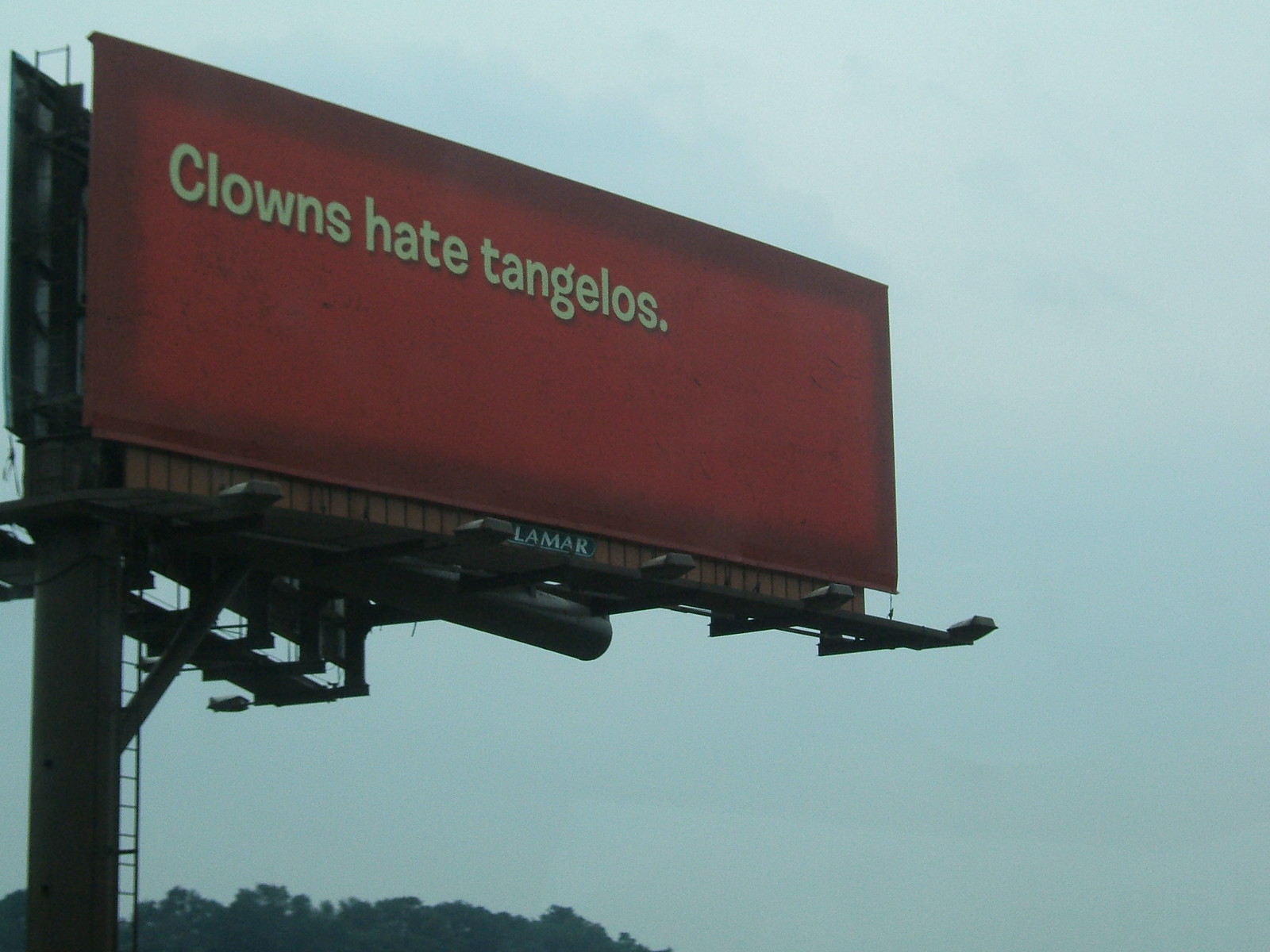The image depicts a prominent red billboard mounted on a thick pole that extends vertically from the bottom to nearly the top of the frame. The billboard's bold red background features the quirky text "Clowns Hate Tangelos" written in a white or slightly yellowish font. Wooden slats are visible at the base of the billboard, providing structural support. The scene's foreground includes the tops of lush green trees, their foliage adding a natural contrast to the artificial structure. The background is dominated by a light blue, whitish sky that enhances the color palette of the image. Both the front and rear sections of the billboard exhibit a series of wooden slats, further emphasizing its sturdy construction.